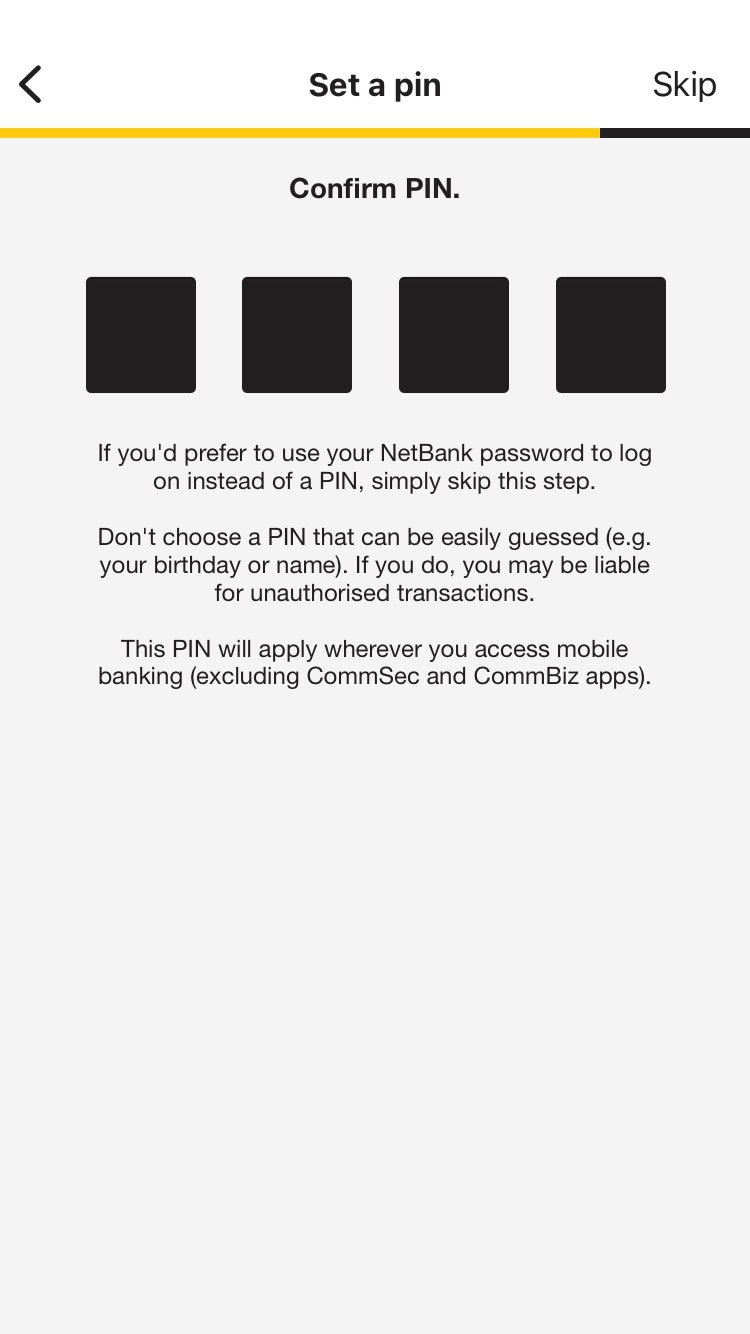The image displays a vertically oriented mobile device screenshot with a "Set a PIN" screen. At the top of the screen, there is a white bar containing black text that reads "Set a PIN." On the right side of this bar, there is a "Skip" option, and on the left side, there is a back arrow. Below this, a progress bar appears, primarily colored yellowish-gold, with a small portion in black on the right end.

Beneath the progress bar, the background transitions to light gray. Centered at the top of this section, bold text with capitalized letters reads "Confirm PIN." Below this heading, there are four equally spaced black boxes that are slightly taller than they are wide, creating a rectangular yet nearly square appearance.

Further down, three blocks of instructional text in black provide guidance:
1. "If you prefer to use your NetBank password to log on instead of a PIN, simply skip this step."
2. "Don't choose a PIN that can be easily guessed, e.g. your birthdate or name. If you do, you may be liable for unauthorized transactions."
3. "This PIN will apply wherever you access mobile banking, excluding ComSec and ComBiz apps."